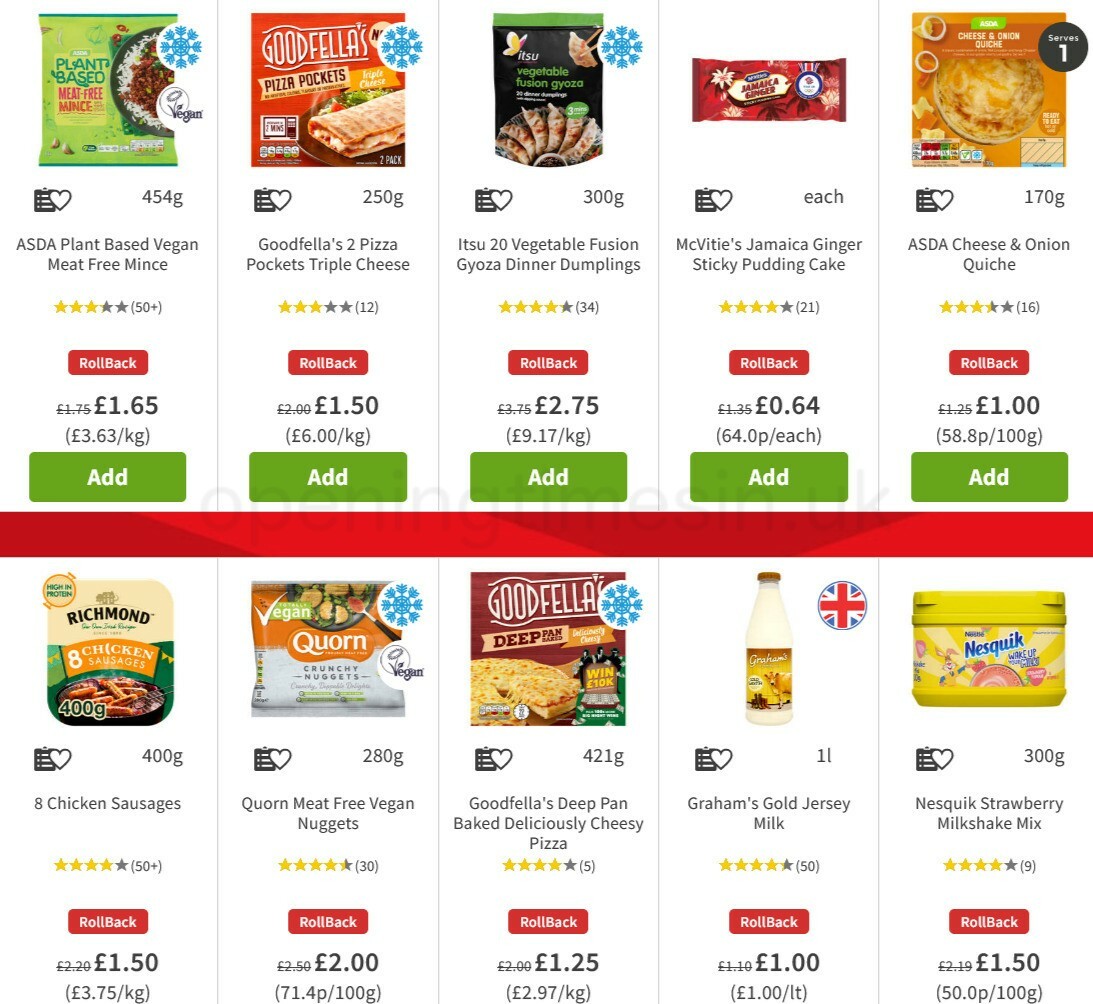### Detailed Caption:

In this meticulously organized image with a white background, we see a neat arrangement of various food items presented in small boxes. Each box is separated by blue lines in the first row and a bold red line between rows, with additional blue lines between the boxes in the second row. The following items are listed:

#### First Row:
1. **ASDA Plant-Based Vegan Meat-Free Mince**: This product features a "Red Rollback" label, priced at $1.65, accompanied by a green "Add" button.
2. **Goodfellas Two Pizza Pockets Triple Cheese**: Displayed with a three-star rating, this item also showcases a rollback price of $1.50 and a green "Add" button.
3. **Itsu 20 Vegetable Fusion Gyoza Thinner Dumplings**: Boasting a four-star rating, this product is priced at $2.75 with a rollback and a green "Add" button.
4. **McVitie's Jamaica Ginger Sticky Pudding Cake**: This cake has a four-star rating and a rollback price of $0.64 accompanied by a green "Add" button.
5. **ASDA Cheese and Onion Quiche**: With a three and a half star rating, priced at $1.00, and features a rollback and a green "Add" button.

#### Second Row (below the red line):
6. **8 Chicken Sausages**: Rated four stars with a rollback price of $1.50 and a green "Add" button.
7. **Quorn Meat-Free Vegan Nuggets**: This product showcases a four and a half-star rating, rollback price of $2.00, and includes a green "Add" button.
8. **Goodfellas Deep Pan Baked Deliciously Cheesy Pizza**: Currently has a four-star rating, a rollback price of $1.25, and a green "Add" button.
9. **Graham's Gold Jersey Milk**: Offered with a rollback price of $1.00 and a green "Add" button.
10. **Nesquik Strawberry Milkshake Mix**: Featuring a four-star rating and a rollback price of $1.50 with a green "Add" button.

Each product square elegantly contains a small black and white paper icon with a white heart symbol, adding to the visual coherence of the display.